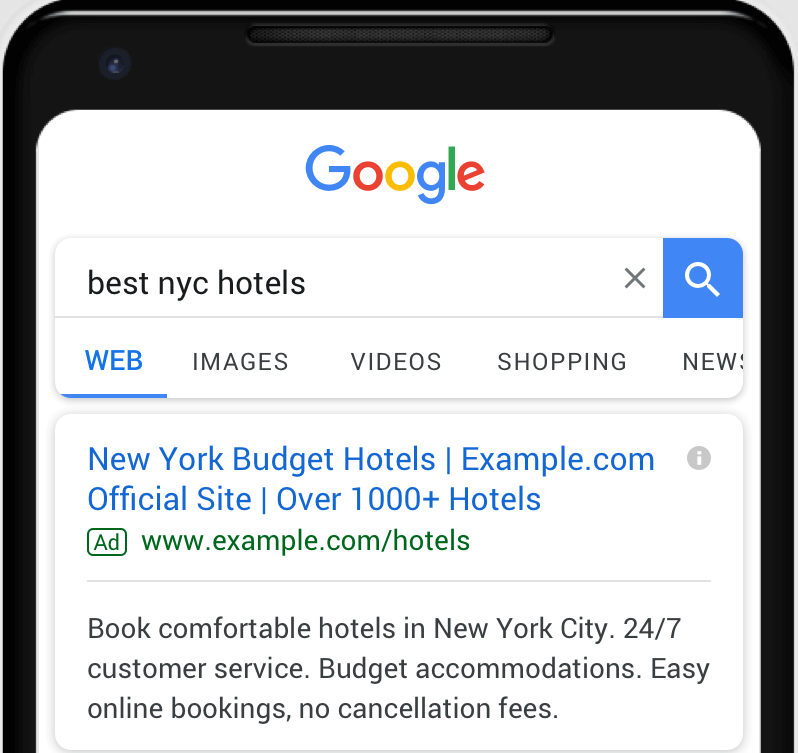The image shows the upper portion of a smartphone, prominently displaying a Google search interface. The phone’s top black border is visible, along with a small, left-aligned front camera and a long, narrow speaker grille centered at the top. 

The smartphone's screen features a Google search page with a white background. At the top-center, the colorful Google logo is displayed. Just below the logo, a search query for "best NYC hotels" is typed in the search bar. To the right of the search text is a gray 'X' icon, and next to it, a blue magnifying glass icon, signifying the search button. 

Beneath the search bar are several tabs labeled: "Web," "Images," "Videos," "Shopping," and a partially visible "News" tab. The initial search results include an advertisement for New York budget hotels, indicating it's from Google.com, the official site. The ad mentions that there are over 1,000 hotels available and highlights features such as bookable comfortable hotels in New York City, 24/7 customer service, budget accommodations, easy online booking, and no cancellation fees.